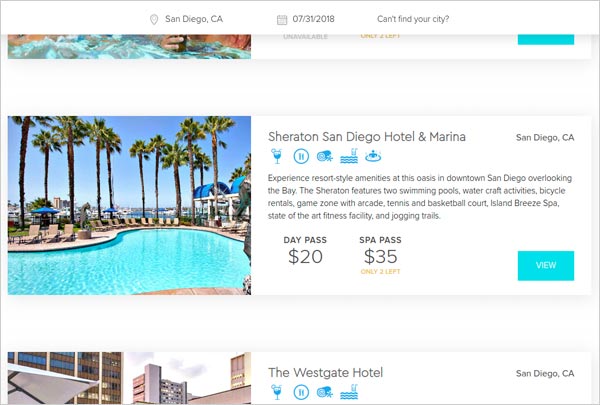**Screenshot from Travel Website: Hotel Details in San Diego, California**

This image captures a section from a travel website featuring prices and descriptions of various hotels. At the top center, the text reads "San Diego, California, 07/31/2018" accompanied by a calendar icon to the left. Below, the site prompts, "Can't Find Your City?"

In the center of the page, there is detailed information about the Sheraton San Diego Hotel and Marina in San Diego, California. On the left side, an image showcases the hotel's swimming pool surrounded by a concrete area, dotted with lounge chairs and framed by palm trees, creating a serene and inviting atmosphere.

The accompanying text describes the hotel's array of amenities: "Experience resort-style amenities at this oasis in downtown San Diego overlooking the bay. The Sheraton features two swimming pools, watercraft activities, bicycle rentals, game zone with arcade, tennis and basketball court, Island Breeze Spa, state-of-the-art fitness facility, and jogging trails."

Additional pricing information includes a day pass for $20 and a spa pass for $35, with the note that only three passes remain available. A prominent blue button to the right labeled "View" invites users to explore more details or make a booking.